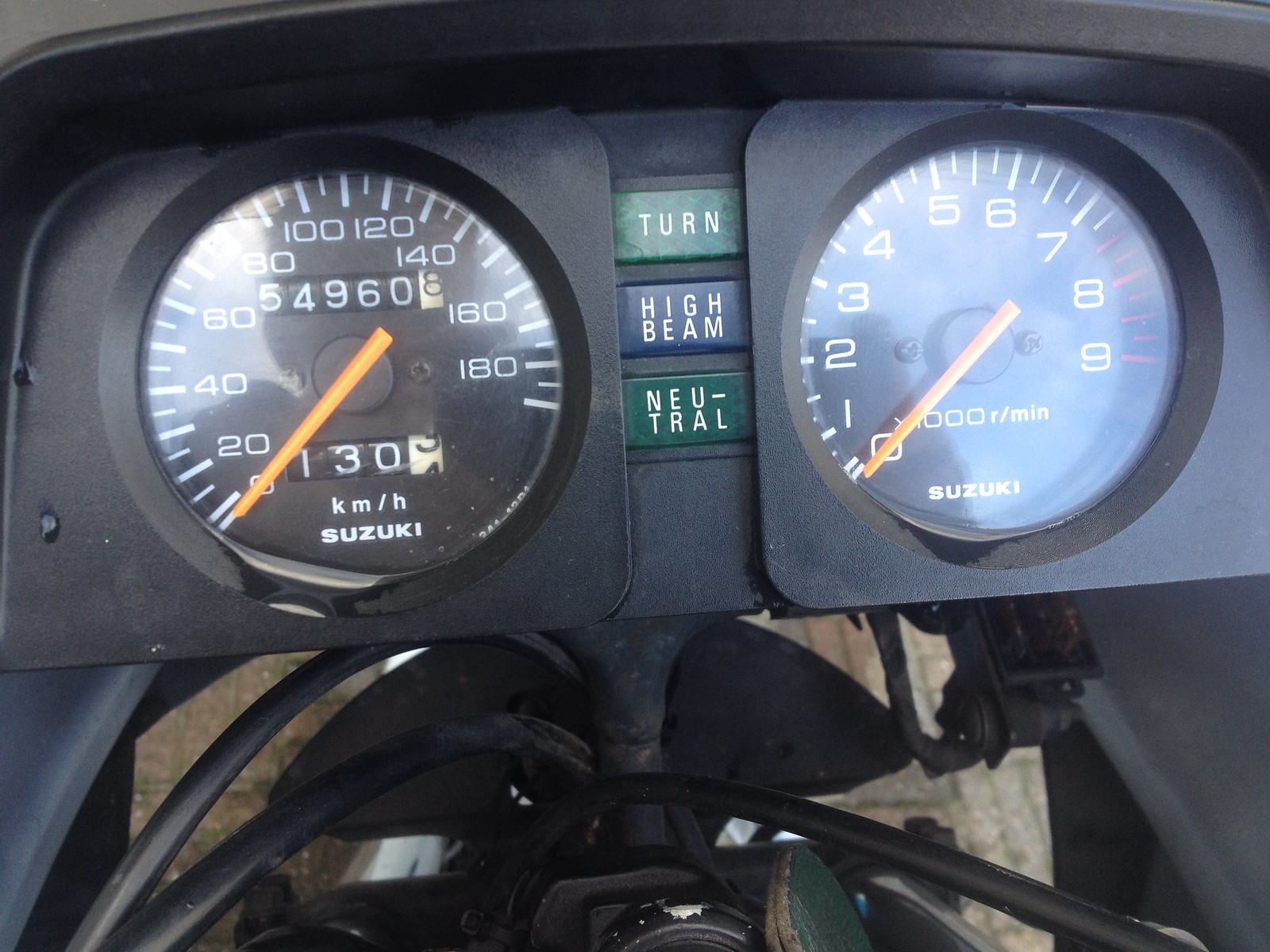A detailed close-up of a vehicle's dashboard reveals a sophisticated setup with various gauges and indicators. Central to the image are two prominent dials. The left dial, marked with "Suzuki," features a speedometer ranging from 0 to 200 kilometers per hour, with a smaller "130" km/h indicator within the dial. An orange needle points to 0 km/h, suggesting the vehicle is stationary. Below this, an odometer reads "54960," with an additional trip meter displaying "0.8" in a white-trimmed section.

In the center, nestled between the dials, there's an arrow slot housing three buttons labeled "Turn," "High Beam," and "Neutral." The "Turn" and "Neutral" buttons have a green-grey background with white text, while the "High Beam" button stands out with a dark blue background and white text.

To the right, the tachometer indicates engine speed, labeled "Revs per Minute," spanning from 1 to 9 with an orange pointer. This dial also bears the Suzuki logo.

The dashboard is set against a black background, possibly composed of a blackish-blue material. Various pipes and mechanical components are visible beneath the gauges, adding to the industrial aesthetic. A wooden backing is discernible towards the rear of the setup, though the specific vehicle type remains unclear.